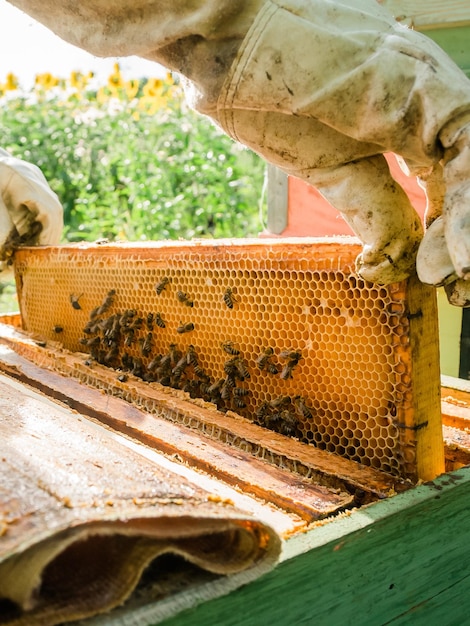A detailed photograph captures a beekeeper in action, identified by their heavy-duty, dirty white gloves, which are visible from the upper left and middle left of the image as they lift a rectangular frame laden with honeycomb and a swarm of bees. The honeycomb, featuring a netted appearance on its underside, is teeming with approximately 20 to 30 bees and is positioned centrally within the frame. A hint of greenery painted wood is noticeable in the lower right corner, suggesting the process is taking place over a beekeeping box. The background is filled with tall green trees or bushes adorned with yellow flowers, and a cluster of sunflowers can be seen standing tall in the top left of the photo. The colors present in the image include dark green, light green, off white, yellow, brown, black, and a touch of pink. The scene is set in an outdoor, likely farm or open field environment, bathed in daylight.